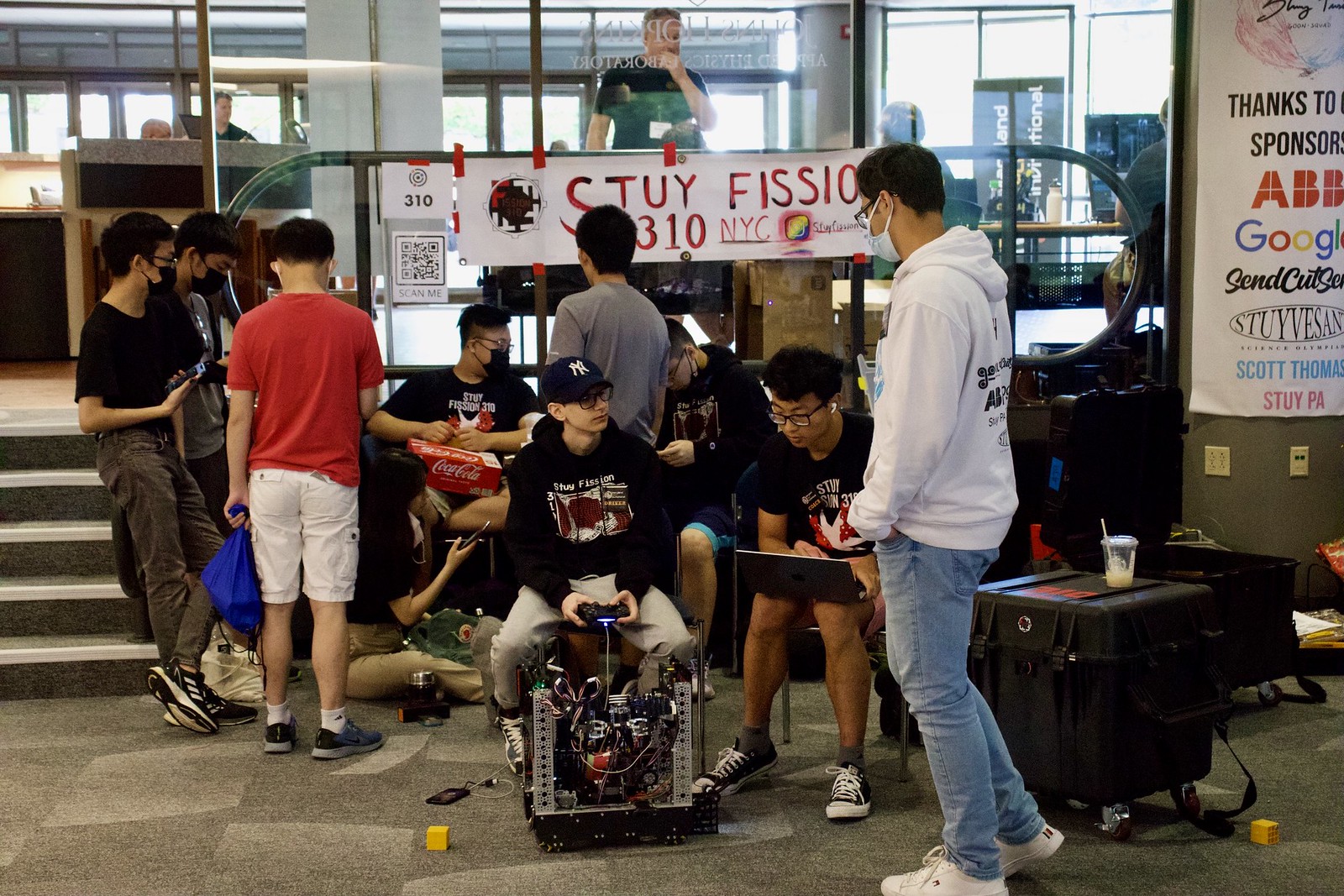In a full-color, indoor photograph taken during the daytime, a group of high school students, predominantly Asian males, are engrossed in an engineering project involving the construction of a remote-control robot, likely for a competitive robot fighting league. The scene is set in a spacious room with a carpeted floor and several windows allowing light to stream in. There are approximately eight or nine students, some wearing COVID masks. The focal point is a student in the center, sitting with a controller in his hand, connected to an exposed mechanical device on the floor. Beside him, another student with a laptop on his knees appears to be coordinating efforts with the controller operator. 

In the background, a banner on the upper right corner attached to a brown post reads "Thanks to our sponsors," listing several entities including ABB, Google, and Stuyvesant, with Scott Thomas and Stuy PA in blue letters towards the bottom. A man in blue jeans and a white hoodie with a COVID mask stands to the right, while another youth wearing a New York Yankees cap and a dark sweatshirt sits on an automated vehicle, hands on the steering wheel. Steps on the left lead to a second floor, which also features a banner with the red lettering "STUY FISSION, NEW YORK CITY." Among the background detritus is a case of Coca-Cola, held by one of the students seated further back. The whole scene is a hive of focused activity, exemplifying youthful ingenuity and collaboration.